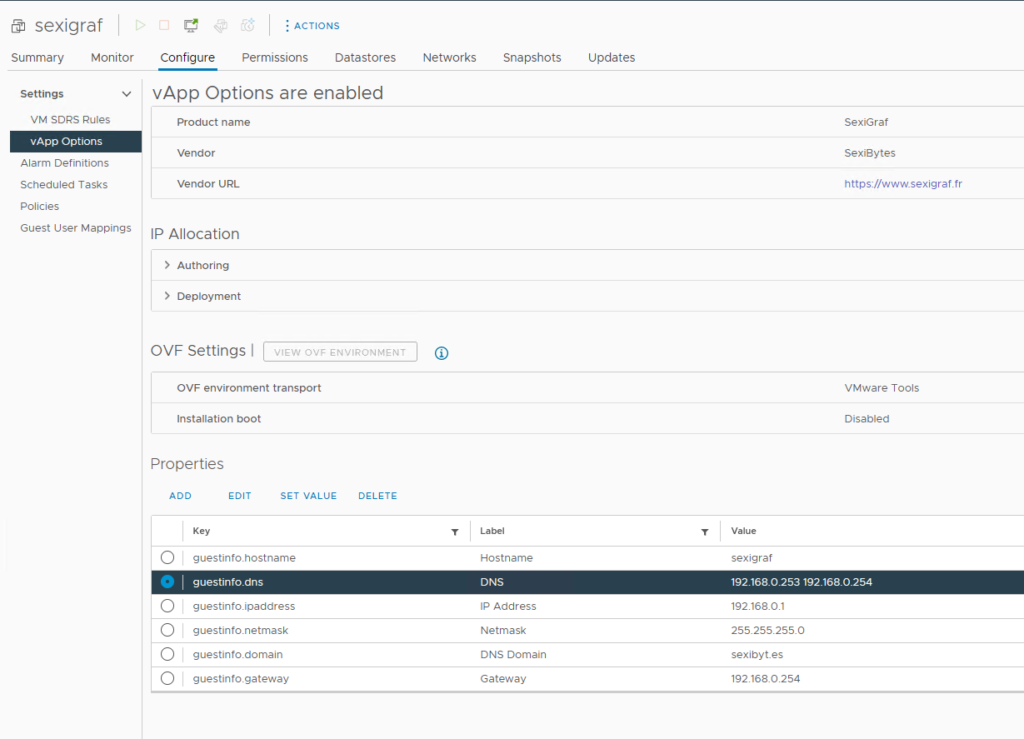This screenshot captures a detailed view of a web interface from SEXIGRAF, a monitoring and configuration tool. Upon closer inspection, here is a descriptive breakdown:

- **Header Information**:
  - **Top Left Corner**: The title "SEXIGRAF" is prominently displayed.
  - **Menu Options Below the Header**: A horizontal navigation bar contains various options including:
    - Summary
    - Monitor
    - Configure (currently selected)
    - Permissions
    - Data Stores
    - Networks
    - Snapshots
    - Updates
  
- **Left-Side Vertical Menu**: This menu lists several configuration categories with the "V-App Options" selected:
  - Settings
  - VMS DRS Rules
  - V-App Options
  - Alarm Definitions
  - Scheduled Tasks
  - Policies
  - Guest User Mappings
  
- **Main Content Area**:
  - **Highlighted Section**: "V-App Options are enabled"
  - **Product Information**:
    - **Product Name**: SEXIGRAF
    - **Vendor**: SEXIGRAF, SEXIBYTES
    - **Vendor URL**: [https://www.sexigraf.fr](https://www.sexigraf.fr)
  - **IP Allocation and Configuration Settings**:
    - **GuestInfo.HostName**: SEXIGRAF
    - **GuestInfo.DNS**: 192.168.0.253, 192.168.0.254
    - **GuestInfo.IPAddress**: 192.168.0.1
    - **GuestInfo.NetMask**: 255.255.255.0
    - **GuestInfo.Domain**: SEXIBYT.ES
    - **GuestInfo.Gateway**: 192.168.0.254
  - **Additional Options and Actions**:
    - Authoring
    - Deployment
    - OVF Settings
    - OVF Environment Transport
    - VMware Tools
    - Installation Boot (option to disable)
    - Properties section with options to Add, Edit, Set Value, or Delete configurations.

This image illustrates the SEXIGRAF interface, demonstrating its extensive array of configurable options catered to network and system administrators for efficient system management.